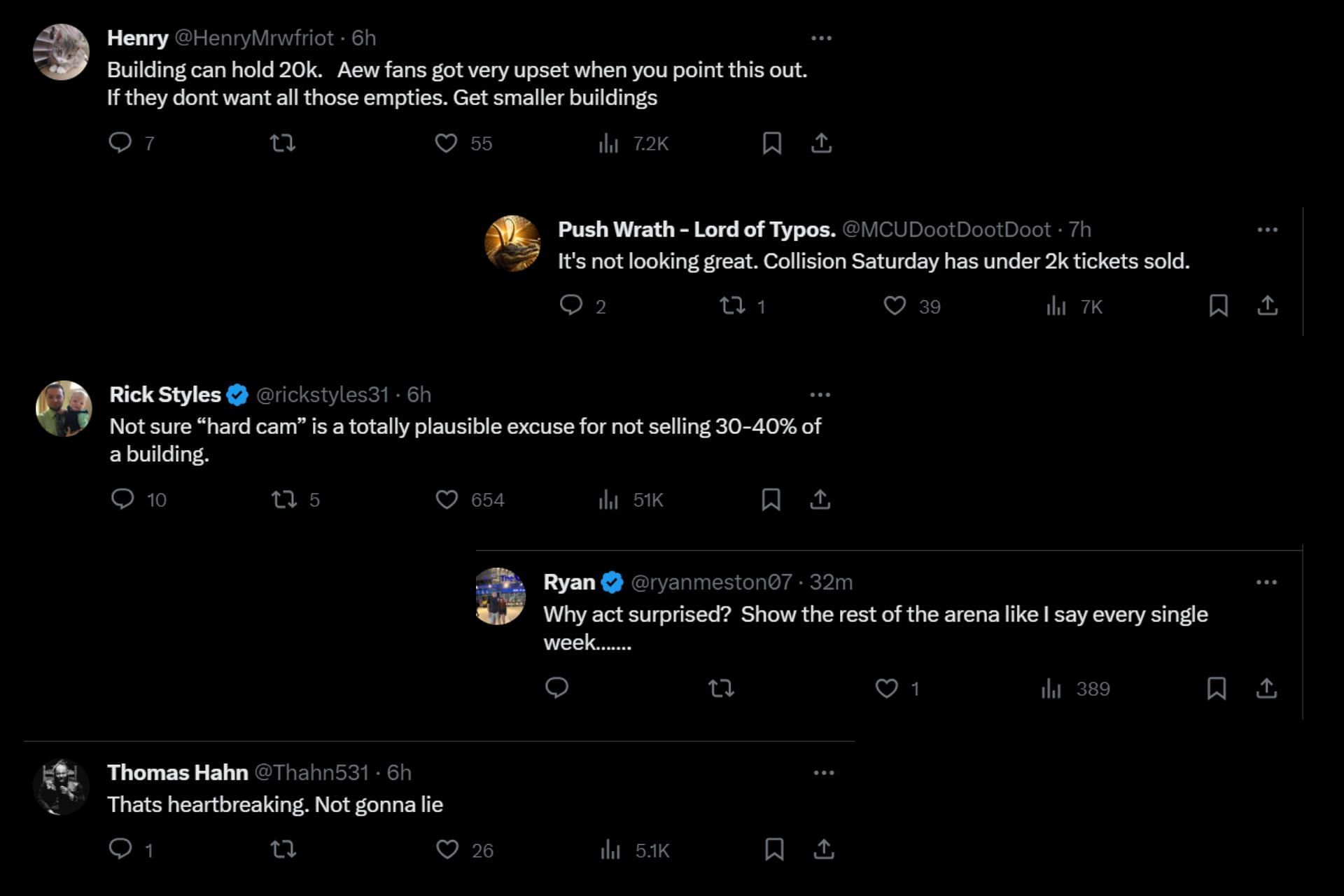The image depicts an edited compilation of five Twitter screenshots, arranged in an alternating left-right pattern against a dark mode background. Each tweet comments on a similar topic, critiquing the attendance and ticket sales of an AEW event.

1. **Henry (@henrymrwfriot)**: "Building can hold 20k. AEW fans get very upset when you point this out. If they don't want all those empties, get smaller buildings."
   
2. **Pushwrath-lordoftypos (@mcudootdootdoot)**: "It's not looking great. Collision Saturday has under 2k tickets sold."

3. **Rick Stiles (@rickstiles31, verified)**: "'Not sure' is a totally plausible excuse for not selling 30 to 40 percent of a building."

4. **Ryan (@ryanmeston07, verified)**: "Why act surprised? Show the rest of the arena like I say every single week........"

5. **Thomas Han (@thanhan531)**: "That's heartbreaking. Not going to lie."

Each of these tweets, expressing disappointment and concern, highlights the issues surrounding event ticket sales and venue capacity, demonstrating a collective sentiment among users about the challenges faced by AEW.